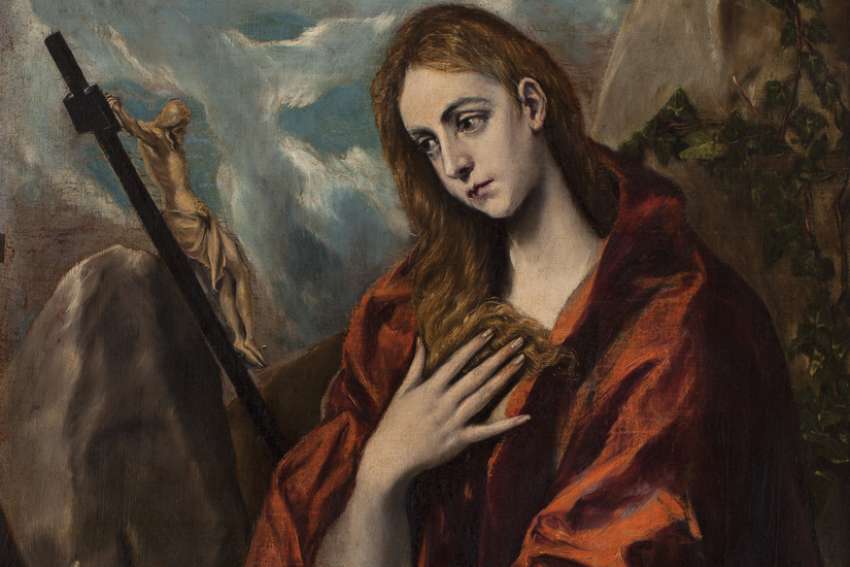This painting, likely an oil painting, depicts a solemn religious scene. A fair-skinned woman with long, reddish-brown or ginger-colored hair stands on the right side. She is dressed in a red robe or cloak, with her right hand pressed to her chest, partially covering her hair. Her gaze is directed downward, imparting a sense of sorrow or contemplation. To her left, a small figure of Jesus is seen crucified on a wooden cross, which leans against a massive rock. The background features stormy, grayish-blue clouds, framing an almost angelic outline in the sky. There are also distant mountains, greenery, and trees or ivy behind the woman. The painting itself is a little wider than it is tall, suggesting a landscape orientation.